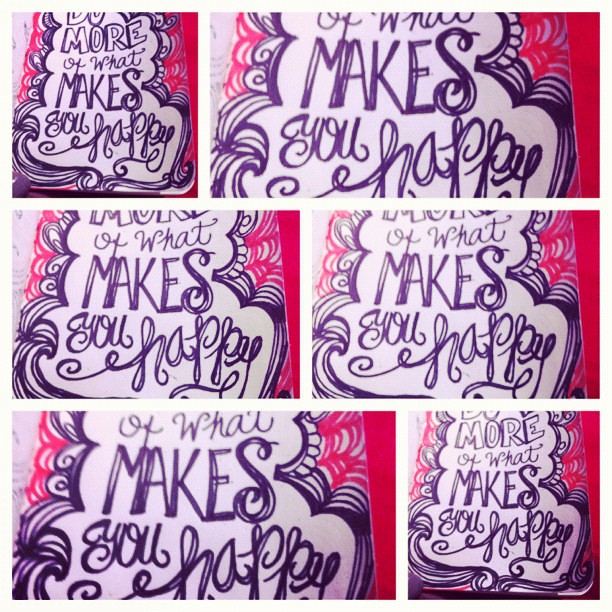The image consists of six differently-sized and cropped photographs of the same artistic representation of a motivational quote. The shared background in all images is pink with a spiderweb-like design subtly highlighted in white. Encasing the central text is a decorative purple ink border, intricate and artistic. The core message, written in a variety of fonts and sizes, reads "Do more of what makes you happy." The phrase is notably structured with "What makes" prominently displayed in large capital letters in the middle, while "you happy" appears at the bottom in elegant cursive. The differing thumbnails include a mix of square and rectangular images arranged in a specific pattern: a square on the top left, a rectangular one besides it on the top right, two squares below them, and at the bottom, one wide rectangle on the left and a narrow rectangle on the right. This composite display, with its vividly designed elements, could easily be part of an art exhibit or designed as a sticker or poster.